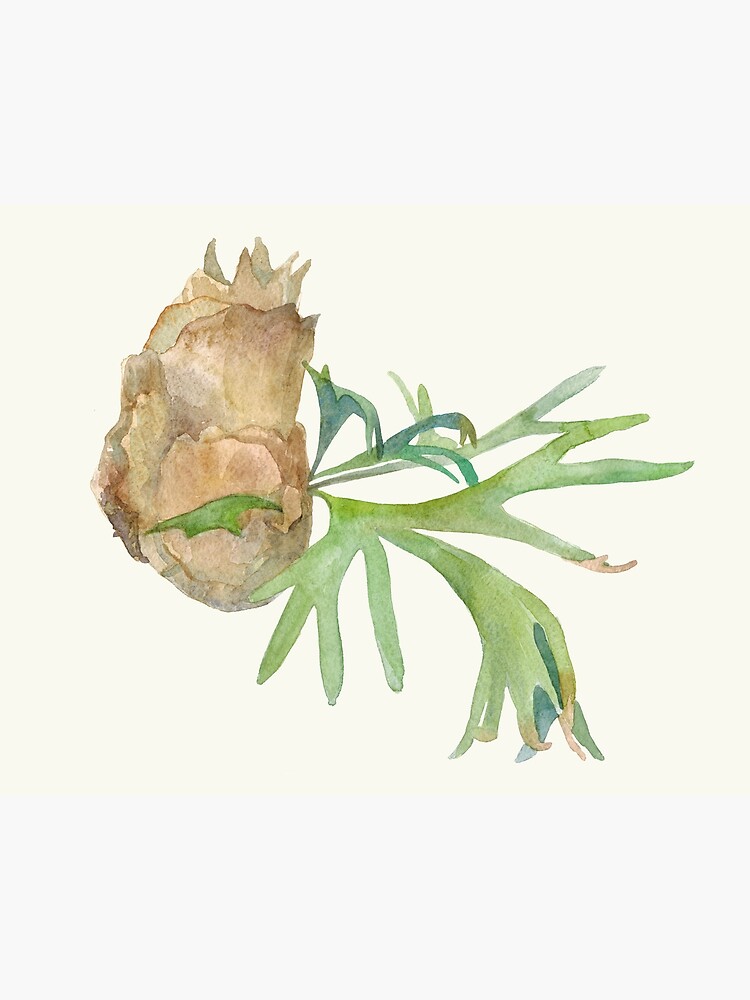The image is a detailed watercolor painting of a plant, capturing a green leaf prominently on the right side, which has some brown tips indicating the leaf is slightly withered. The plant appears to have a brownish root or bulb-like base that resembles an onion, suggesting it's part of a similar family. The artwork uses an off-white canvas as the background, enhancing the vividness of the green and brown colors. The painting conveys a sense of the plant being on the verge of growth or decay, adding a dynamic element to the composition. The scene is indoor, with no additional objects or text, highlighting the plant's intricate details and organic forms.